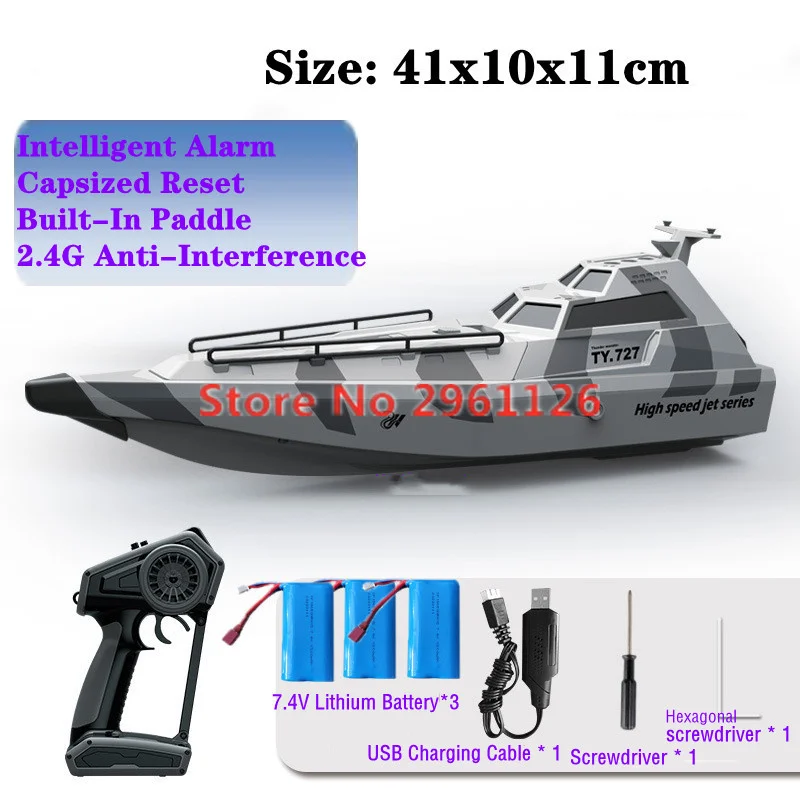The promotional product photo is a detailed diagram showcasing a high-speed jet series remote control (RC) boat in gray and white, with dark gray camouflage-like patterns. The boat, which measures 41 by 10 by 11 centimeters, is labeled with the store number 2961126 in red text. The boat features two converging rails on the top and a small fin at the back, with sealed windows receding towards the rear fin. The boat's nose is black, and "High-Speed Jet Series" and "TY. 727" are painted on its side. 

In the upper left corner of the image, purple text on a blue background highlights the features: intelligent alarm, capsize reset, built-in paddle, and 2.4G anti-interference technology. 

The bottom portion of the image includes a gray square with rounded corners listing the enclosed items: three 7.4-volt lithium batteries, a USB charging cable, a screwdriver, and a hexagonal screwdriver (Allen wrench). Additionally, an intelligent alarm resembling a pistol grip with a wheel dial and trigger is displayed, with the trigger likely serving as the brake and the wheel for forward and backward movement.